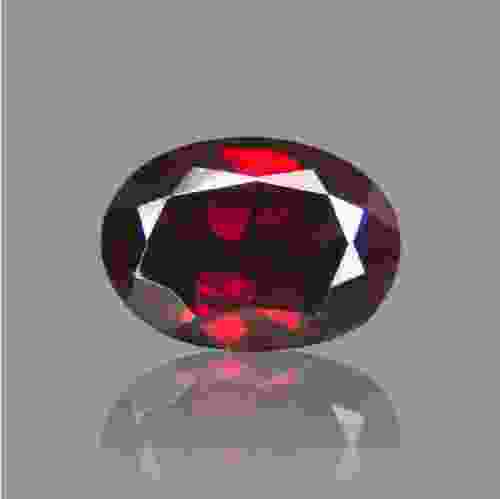The image features a digitally created, low-resolution depiction of what appears to be a gemstone, centrally positioned against a plain, gray background. This gemstone closely resembles a ruby or garnet, characterized by its deep red hue interspersed with various shades of red, maroon, and almost white highlights that suggest reflections of light. The gem is comprised of multiple triangular facets, giving it a complex, pixelated appearance. Beneath the gemstone, a semi-circular shadow or reflection in muted shades of red and gray can be seen, although it lacks clarity and definition. The absence of text allows the focus to remain solely on the intricately designed, yet pixelated gem, which could easily be part of a digital advertisement, online gallery, or printed media showcasing gemstones.